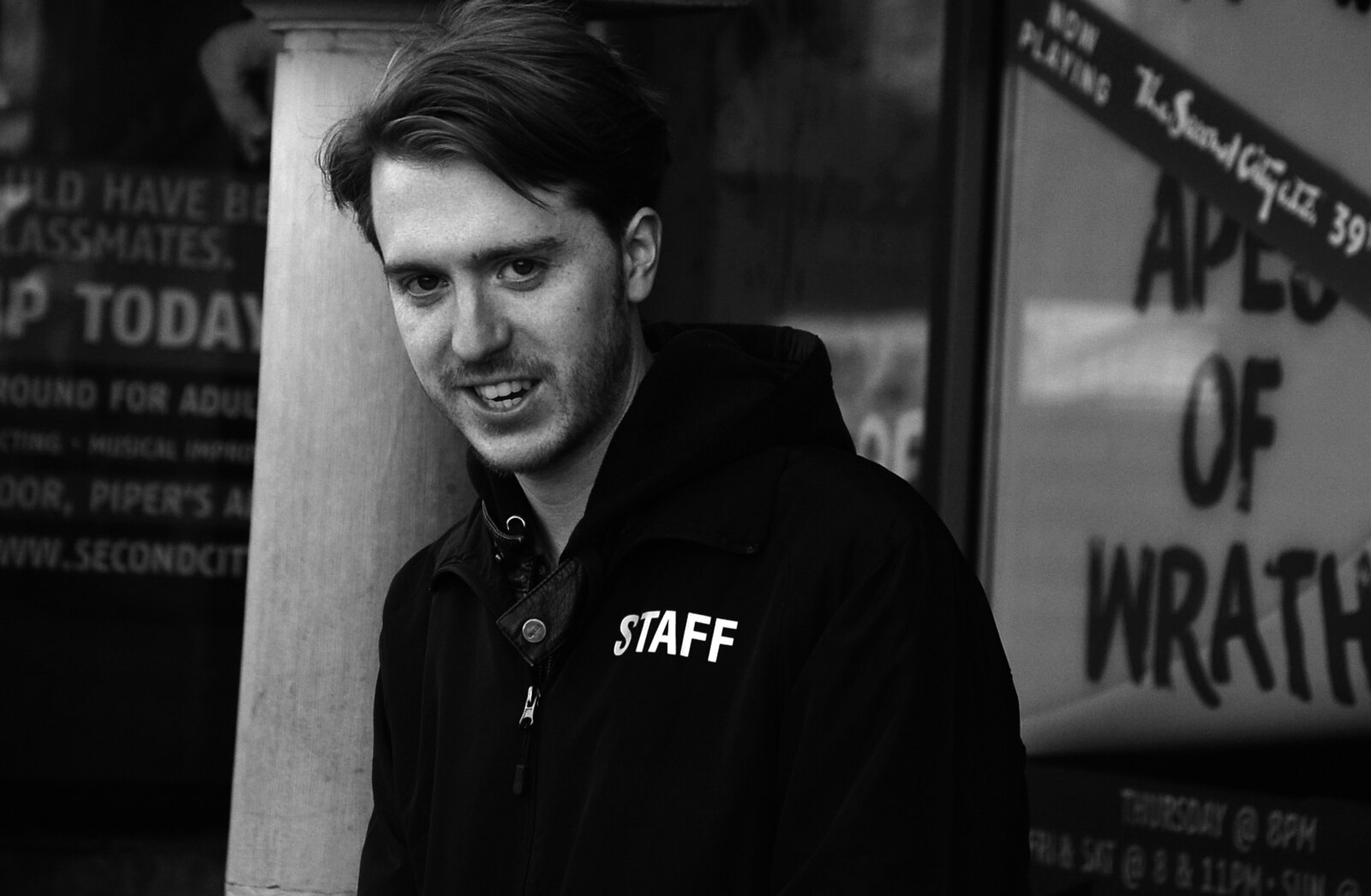This black-and-white photograph captures a young man, likely a staff member at a movie theater, standing next to a column. He is wearing a black hoodie with the word "STAFF" prominently displayed in white letters on the left chest. His hair is short and dark, combed over, and he has a mustache with a bit of a five o'clock shadow. His expression is peculiar, with his mouth open, showing teeth, as if caught mid-sentence or gesture.

In the background, behind him, is a framed movie poster announcing "Apes of Wrath, Thursday at 3 p.m." To the left, there is part of a sign which is partially cut off, displaying some legible text: "have classmates today for adults Piper's" and "www.secondcity.com," hinting at some association with the Second City comedy troupe. The young man stands amid this collage of movie and event posters, creating context and environment for what looks like a casual yet intriguing moment captured outside a bustling venue.